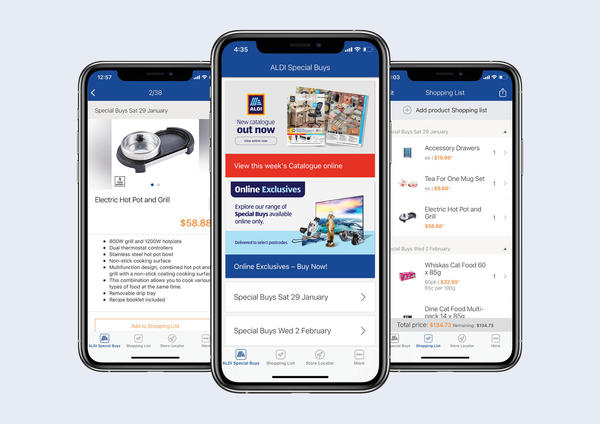The image features a large rectangular backdrop in a light blue-gray hue, adorned with three overlapping smartphone screens arranged horizontally. The central phone screen prominently overlaps the two on its sides.

- **Left Screen:** Displays a product listing for an electric hot pot and grill priced at $58.88. The screen provides the product image but omits detailed product information.

- **Center Screen:** Dominated by the Aldi logo, it announces "Aldi Special Buys" with the tagline "New catalog out now." Adjacent to this announcement is an image of the catalog showing various product images. The text on an orange background encourages readers to "View this week's catalog online." Below this, there's a button labeled "Online Exclusives," accompanied by the text: "Explore our range of special buys available online only." To the side, an image of a large television screen appears, although it is too blurry to distinguish its content. The section concludes with two prominent dates: "Special Buys Saturday 29 January" and "Special Buys Wednesday 2 February" underlined by the phrase "Online Exclusives. Buy Now."

- **Right Screen:** Titled "Shopping List," it enumerates several items, starting with "Accessory drawers" (followed by an indistinct price), "Tea for one mug set" (with an illegible price), and "Electric hot pot and grill" (price unreadable). It continues with two listings of Whiskas cat food, one with a clearly visible price. The screen concludes with a total price at the bottom.

Overall, the image focuses on Aldi’s special promotions and featured products, with an emphasis on the convenience of online shopping and personalized shopping lists.